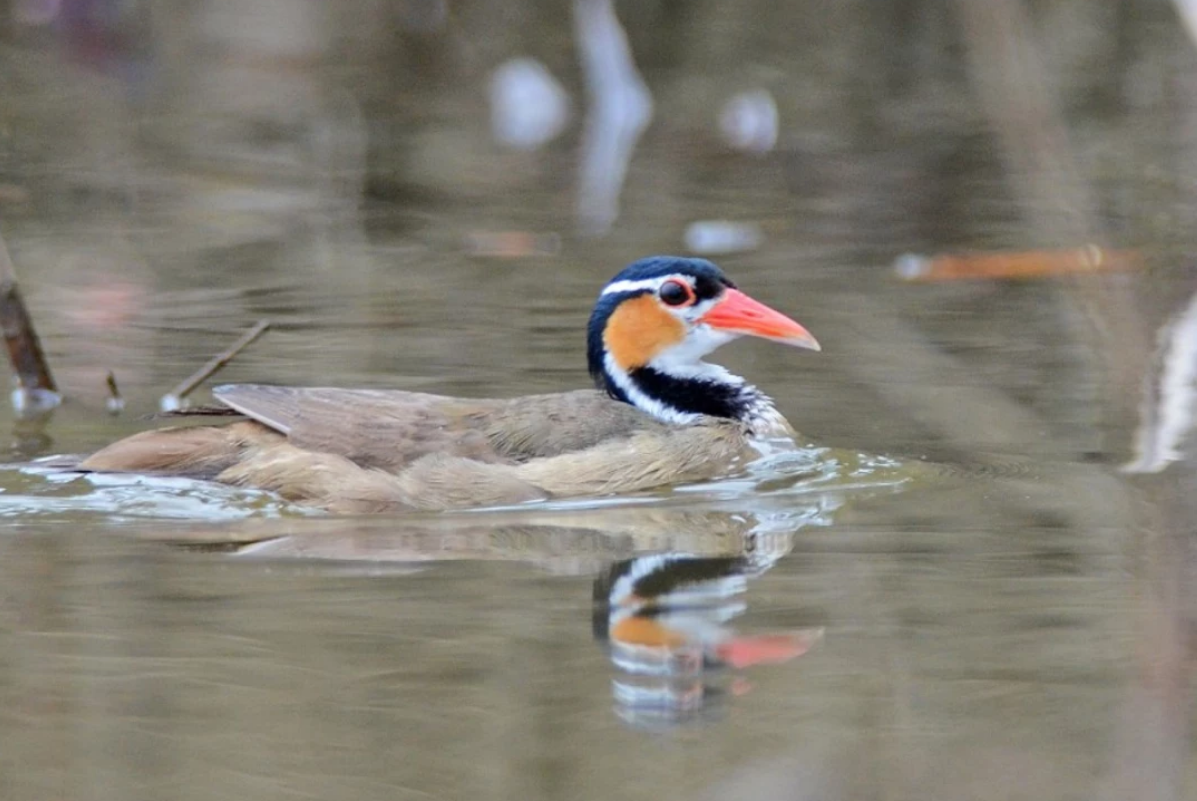The photograph features a striking aquatic bird, swimming and half-submerged in a highly reflective, yellowish body of water. The focus of the image is squarely on the bird, with the blurred background hinting at various trees and vegetation. The bird itself is moving from left to right, presenting its detailed right profile. 

Its plumage is a blend of tan, grey, and light beige on the back and wings, providing a muted contrast to the striking colors of its head and neck. The bird's head is predominantly black, with a distinctive white stripe above its large, black eye. Below the eye, a vibrant orange patch catches the light, while its long, pointed beak is a brilliant orange with a greyish underside. The neck features black and white stripes, adding to its distinctive markings. The water's reflective surface perfectly mirrors the top half of the bird, doubling the visual impact. Overall, this photograph captures the serene yet vivid details of the bird in its natural habitat.